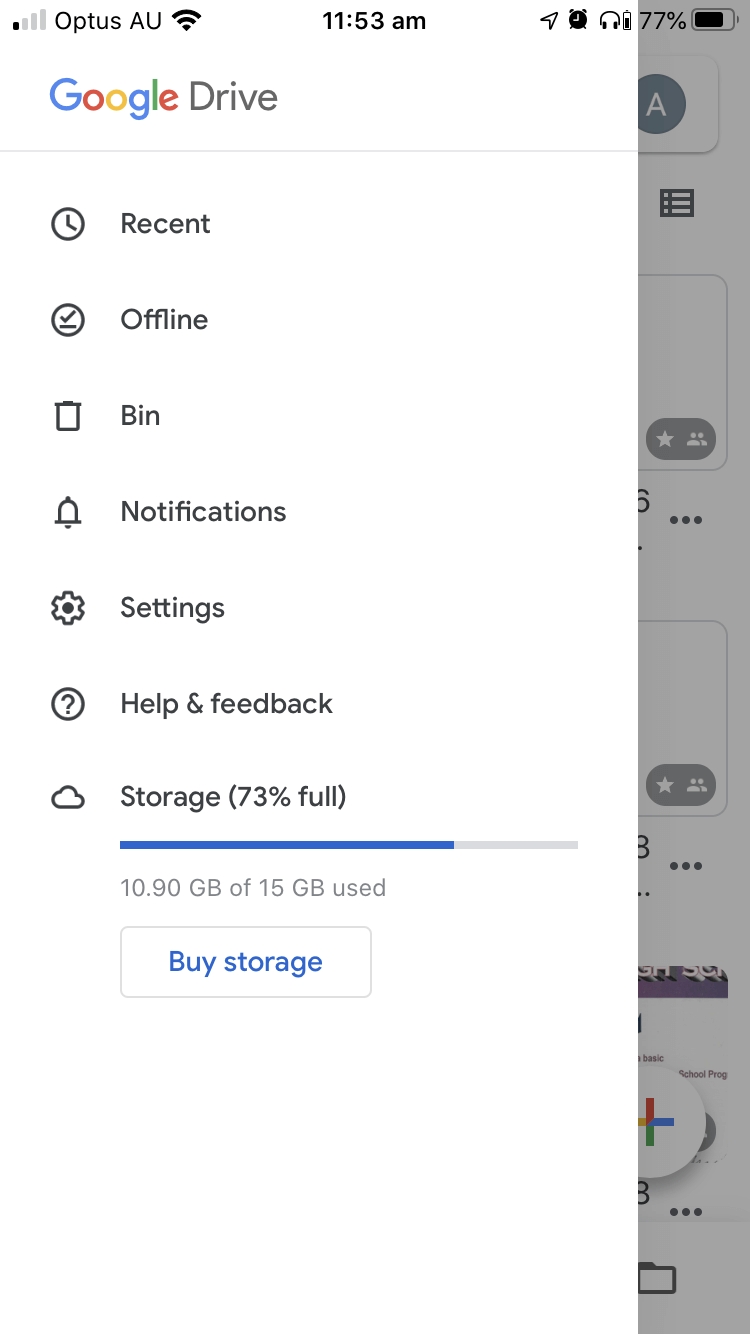Screenshot of a Google Drive interface on a mobile phone. In the upper left corner, the status bar indicates one out of four bars for cellular reception with the label "Optus AU" next to a full Wi-Fi signal icon. The time displayed is 11:53 AM. Below the status bar, the screen shows the Google Drive app, starting with the "Recent" section marked by a clock symbol. A label indicating “Offline” status is displayed with a check mark and a trash icon beside it. Just below, there's a notifications icon followed by the word "Notifications." Further down, a settings gear icon appears with the label "Settings" and a question mark icon labeled "Help & feedback." The storage information is presented next, showing a cloud icon followed by text indicating "Storage 73% full, 10.90 GB of 15 GB used." A blue "Buy storage" button is available below the storage information, all set against a white background with light gray accents.